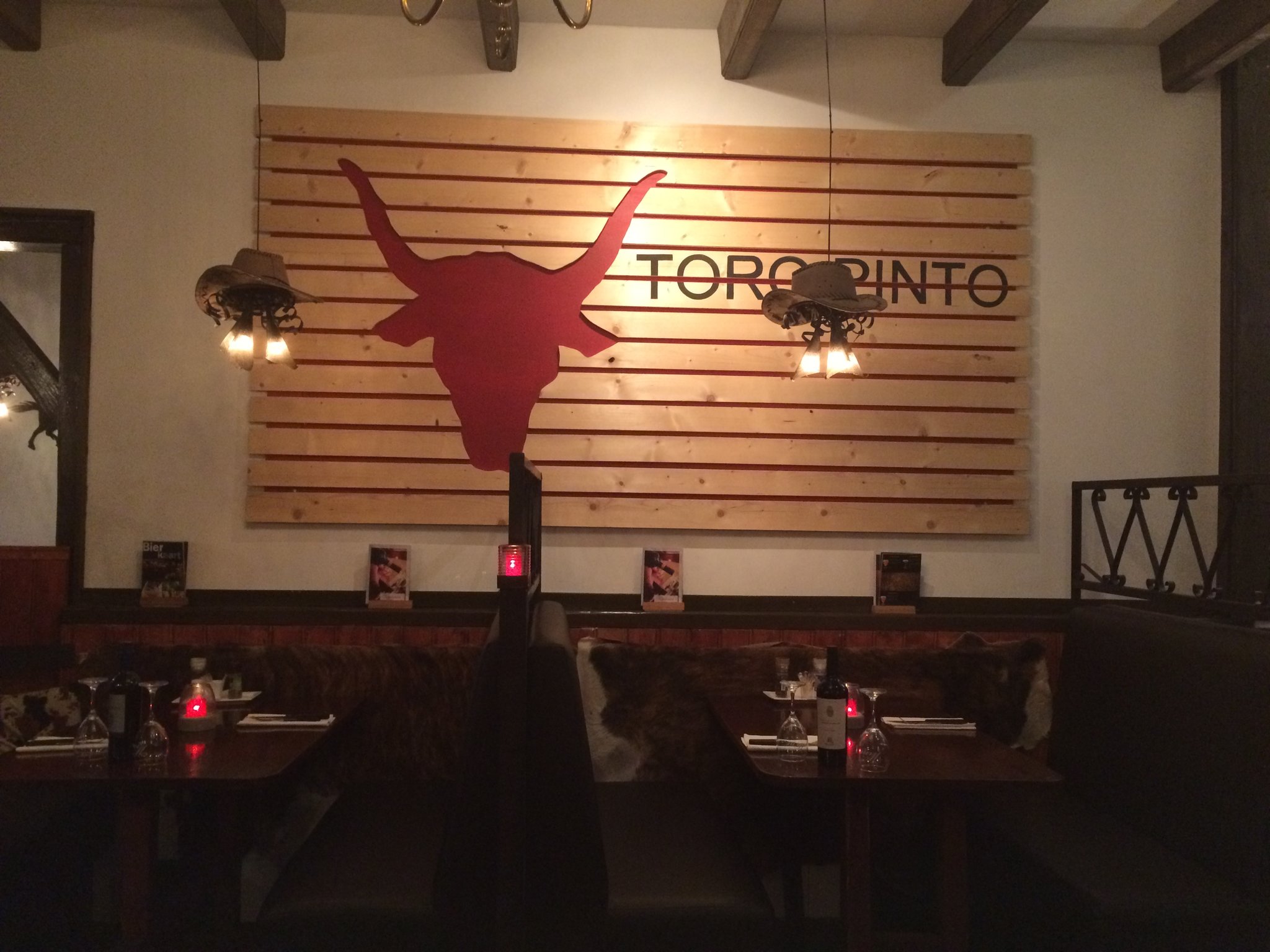This image captures the dimly lit interior of a cozy restaurant named "Toro Pinto." In the foreground, two empty brown booths with padded seating flank wooden tables, each large enough to accommodate four or five people. The tables are elegantly set with napkins, silverware, upside-down wine glasses, and a bottle of wine. A lit candle encased in a red globe adds a warm ambiance to the setting.

In the background, a white wall is adorned with a large wooden sign featuring the silhouette of a bull's head in red, and the words "Toro Pinto" to the right. The letters "O" and "P" are slightly obscured by a unique chandelier that hangs from the ceiling; each of its three lights is stylishly topped with a cowboy hat. The overall decor combines rustic elements with refined touches, creating an inviting and intimate dining atmosphere.